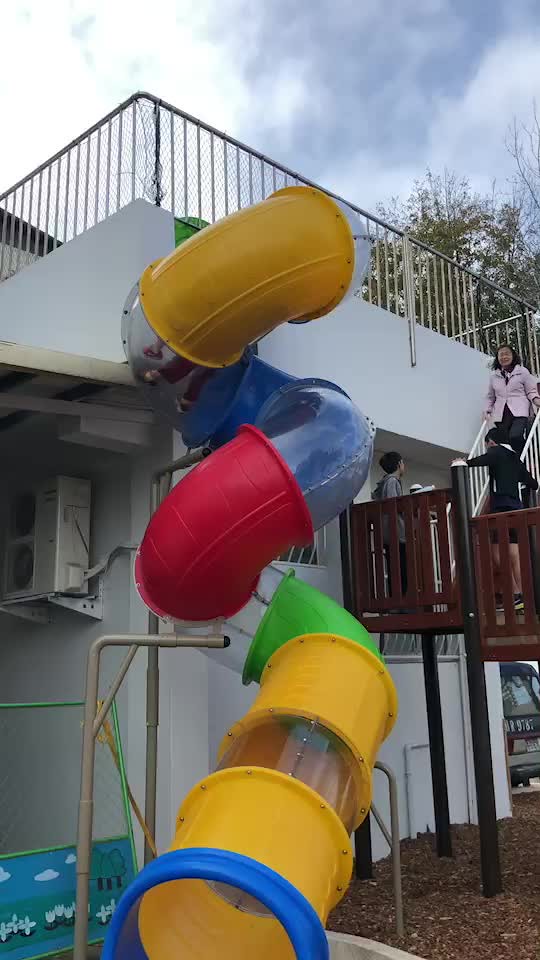This vibrant color photograph, taken outdoors on a partly cloudy day, captures the lively corner of a white stucco building featuring a unique multi-colored, twisty slide similar to those found in McDonald's play places. The slide, with its series of tubes in alternating transparent, yellow, blue, red, and green segments, makes approximately three full rotations as it descends from an upper patio balcony. Adjacent to the slide, a stairway leads both up and down the building, where a woman in a pink jacket and black pants is seen walking down, accompanied by two young boys. The scene is set against a backdrop of a blue sky dotted with clouds, and mulch is visible at the base near the colorful slide, lending a child-friendly atmosphere to the setting. The bottom left corner also features a cartoony, kid-oriented sign, enhancing the playful environment of the scene.